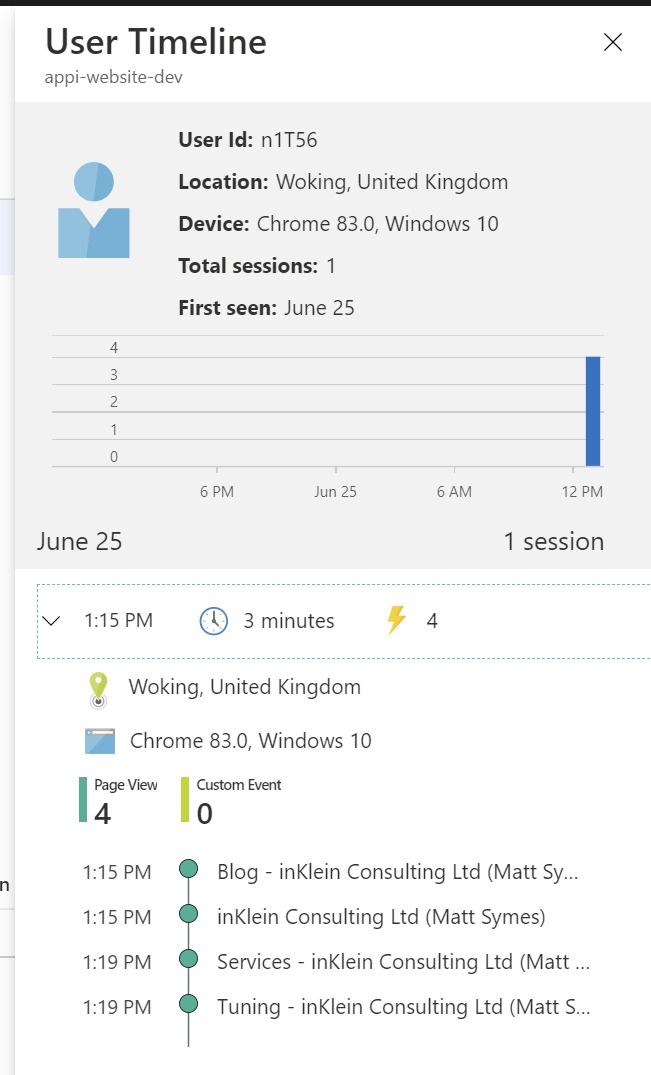### Detailed Image Caption:

At the top of the image, the heading reads "User Timeline," indicating a timeline of a user's activity. Below this heading, the source of the data is described as "Development," with a note that it originates from a website developer.

The main section of the image displays a gray box that contains user information. On the left side of the box, there is a small blue avatar icon. To the right of this icon, the text identifies the user by "User ID: 1256". 

Further details include the location "Woken, United Kingdom" and the device used, which is specified as "Chrome 83 on Windows 10". This user has had a total of one session, with the first recorded activity date being June 25th.

Below this data, a bar graph visually represents this single session, showing activity peaking at 12:00 PM. The bar graph is depicted in blue, extending from zero and peaking at approximately 3.5 units.

Beneath the bar graph, it specifies again "June 25th, 1 session," with a dropdown next to a clock icon. This clock indicates the session lasted for three minutes. Next to a lightning bolt symbol, there is a number 4, suggesting some metric related to activity or performance.

Further down, a green location pin with the text "Woking, United Kingdom" is displayed, followed by device information reiterating "Chrome 83 on Windows 10". The page view and custom event data below show two vertical lines—a darker green line for page views and a lime-green line for custom events, both of which are thickly drawn.

The final section of the image lays out a timeline of specific activities during the user's session:
- At 1:15 PM, the user accessed "Blog Incline Consultant LTD".
- Also at 1:15 PM, there was another access listed as "Incline Consulting with Matt Symes".
- Four minutes later, at 1:19 PM, the user interacted with "Services Incline", again with a reference to Matt Symes.
- Finally, the user accessed "Tuning Incline Consulting with Matt" at an unspecified time shortly after.

This detailed visual data provides a comprehensive look at a user's interaction with a website, breaking down the specifics of their session and activities.